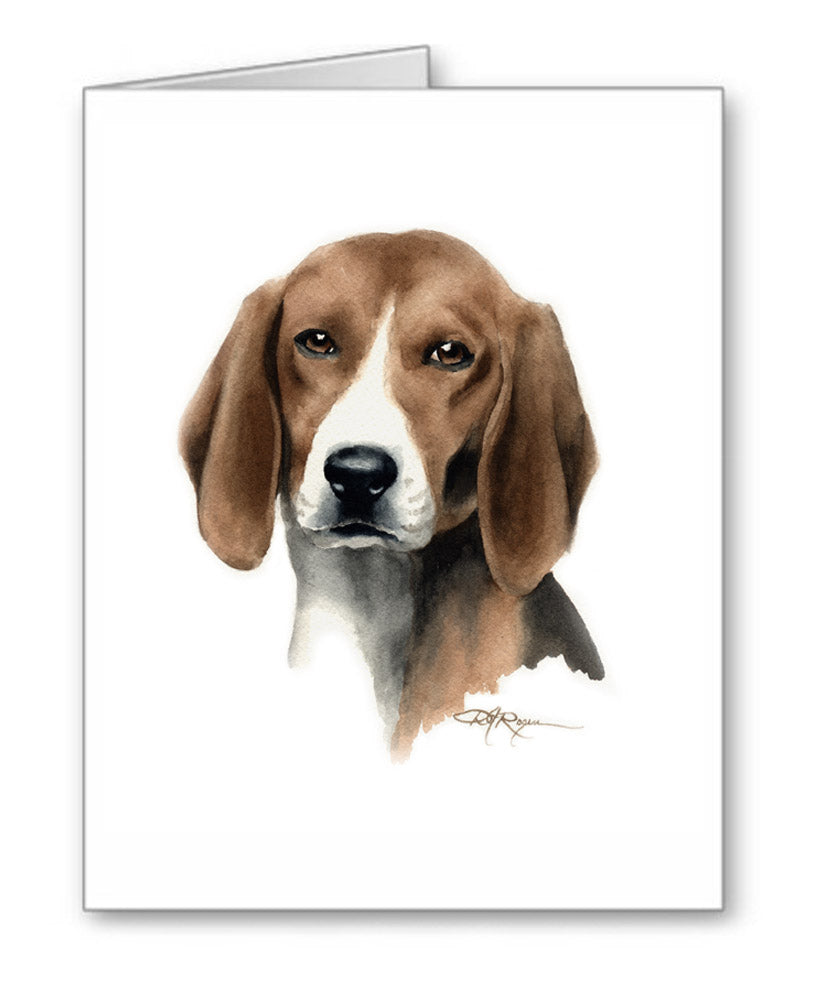The image depicts a digitally rendered greeting card displaying a watercolor-like drawing of a beagle's head and neck against a white background. The card stands open on a white surface, revealing its front in a rectangular, portrait layout, with the longer sides on the left and right. The featured beagle has distinctive brown ears, a white muzzle, a black nose, and expressive brown eyes, staring straight ahead. Its long, floppy ears frame its face, which is marked by a white spot between the eyes running down to its neck. There is a brown cursive artist's signature positioned on the lower right below the dog's head. The card has a grayish-black border, and a small triangular peek at the top suggests its open state, indicating the inner side of the card is not visible. The entire setting emphasizes the minimalist, clean design of the greeting card.